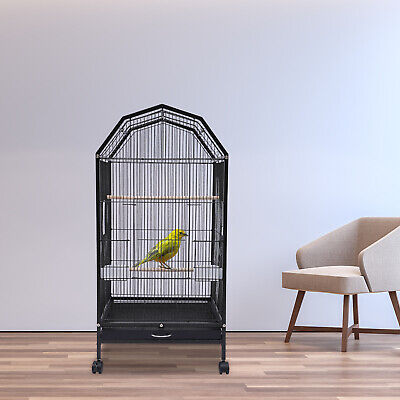The photograph captures a pristine, minimalist-style room characterized by its modern light tan wooden floor and solid white wall. Dominating the right side of the image is a sleek, modern chair with a leather-look finish, featuring a medium-height back and wide, sloped sides set on four legs. Central to the composition is a tall, black wire birdcage, about chin height for most adults, with a pull-out seed tray at its base engraved with an illegible white logo. The cage exhibits a mix of vertical and horizontal bars, forming an arched top and divided into multiple layers, offering ample vertical space for flight. Perched on a white stick in the lower third of the cage is a large, bright yellow parrot with green wings and possibly grayish tail feathers, facing towards the right. The sparse yet thoughtfully arranged elements of the room emphasize a contemporary and uncluttered aesthetic.